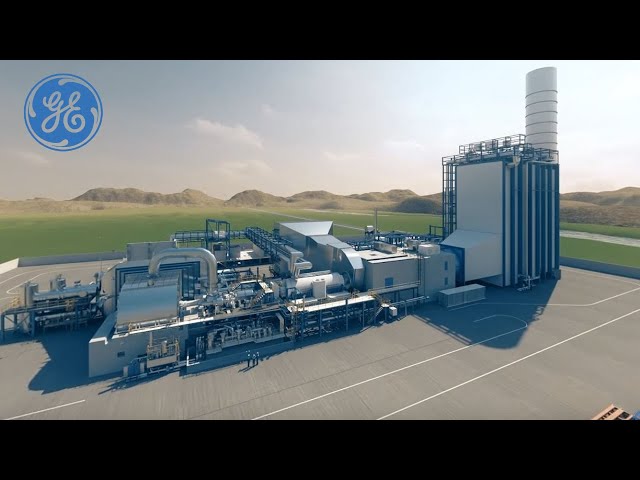The image is a detailed photograph of a large industrial complex, prominently featuring the GE (General Electric) logo in the upper left corner, set inside a blue circle with a wavy border. The complex is set against a backdrop of brown hills and a partly cloudy sky, with a well-maintained green grassy lawn below the hills. The main structure of the complex is predominantly silver and metallic, with various sections differing in size and shape. A noticeable chimney stack rises from the tallest part of the building, making it significantly higher than the other sections. In front of the building, which is situated on a concrete structure marked with white lines, three small figures can be seen conversing, though their details are indistinguishable. The image has black borders at the top and bottom, framing the industrial scene.